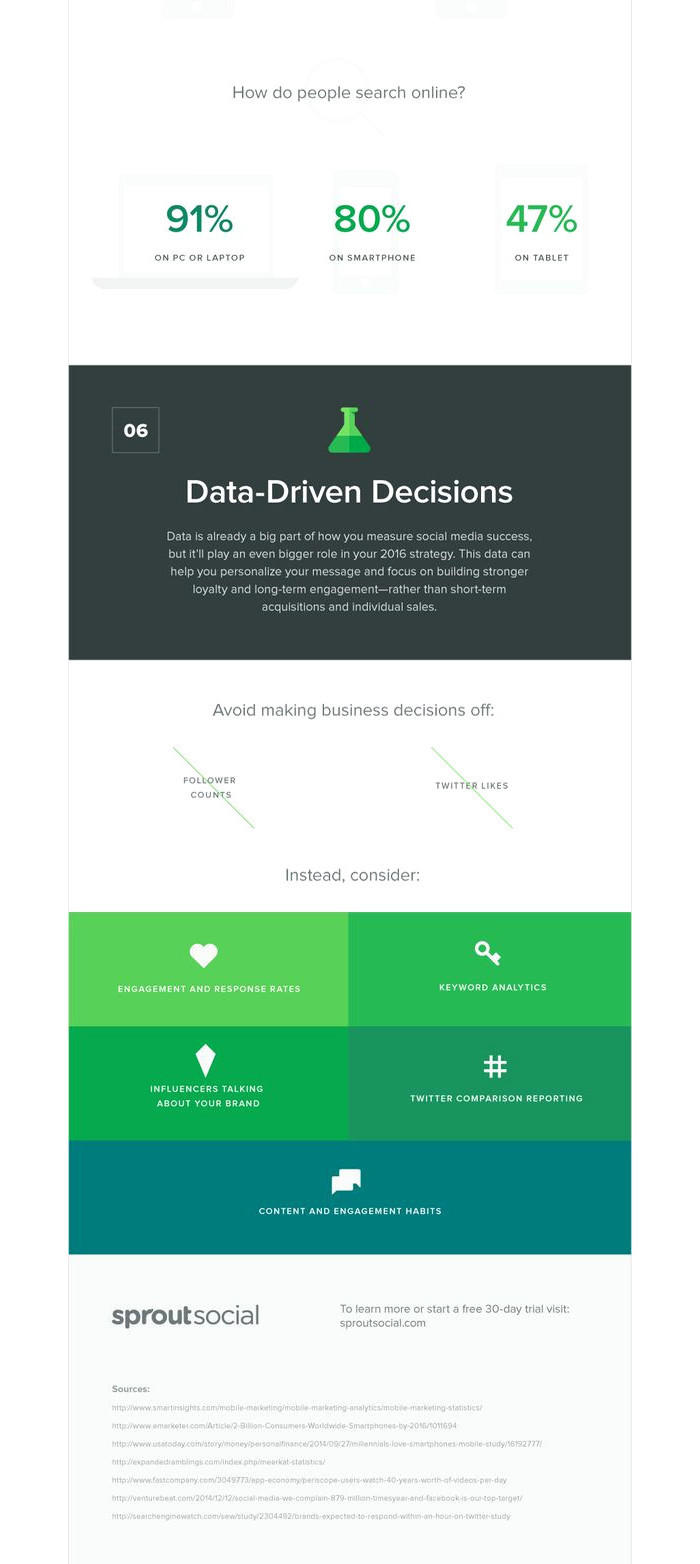In this detailed screenshot, the focus is on how people conduct online searches. Displayed prominently at the top center are three key statistics: 91% of users search via PC or laptop, 80% use smartphones, and 47% utilize tablets. 

Below these percentages, the header "Data-Driven Decisions" introduces a section emphasizing the importance of data in measuring social media success. The text elaborates that while data is already crucial, it will become even more integral to strategies in 2016. Key points include the role of data in personalizing messages and fostering stronger loyalty and long-term engagement, as opposed to solely driving short-term acquisitions and sales.

The following segment advises against making business decisions based on follower counts and Twitter likes. Instead, it suggests considering other metrics, displayed in five small rectangles with text too minuscule to decipher.

At the bottom of the screenshot, the logo "Sprout Social" is visible, accompanied by what appears to be various website link sources. This comprehensive layout underscores the growing importance of data in shaping effective social media strategies.